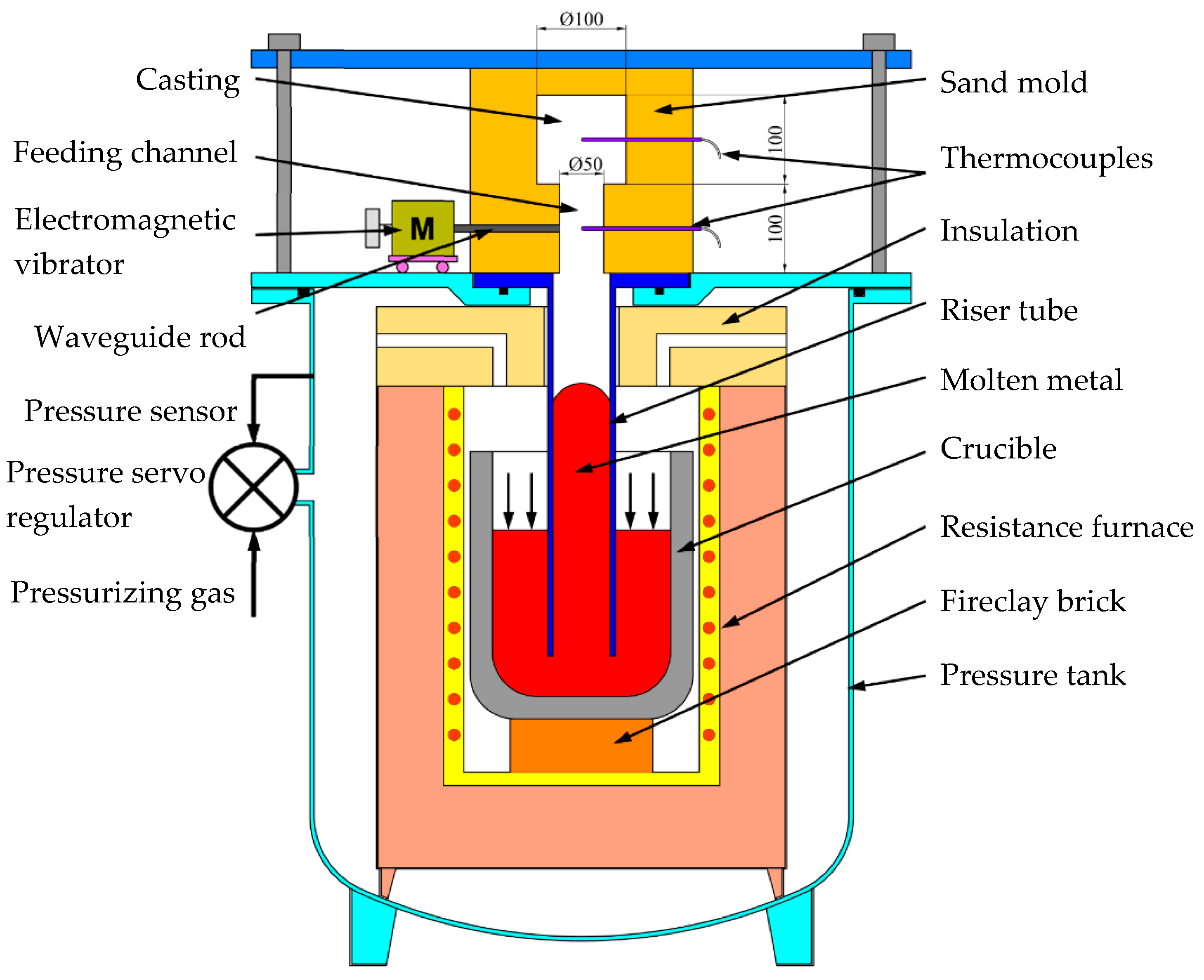The image depicts a detailed diagram of a mechanical device, likely a furnace, set against a white background. At the top, the diagram features a horizontal blue bar, followed by an orange square centrally located below it. Beneath the orange square, two horizontal green bars are positioned one above the other. 

Below these green bars lies a rectangular structure, with its top portion colored yellow and the bottom pink. A central tube extends from the yellow section down into the rectangle, which contains red liquid within. 

The diagram is heavily labeled on both sides with annotations such as casting, feeding channel, sand mold, thermocouples, electromagnetic vibrator, waveguide rod, pressure sensor, servo regulator, pressurizing gas, riser tube, molten metal, crucible, resistance furnace, fireclay brick, and pressure tank. These labels help identify various components and functions of the machine.